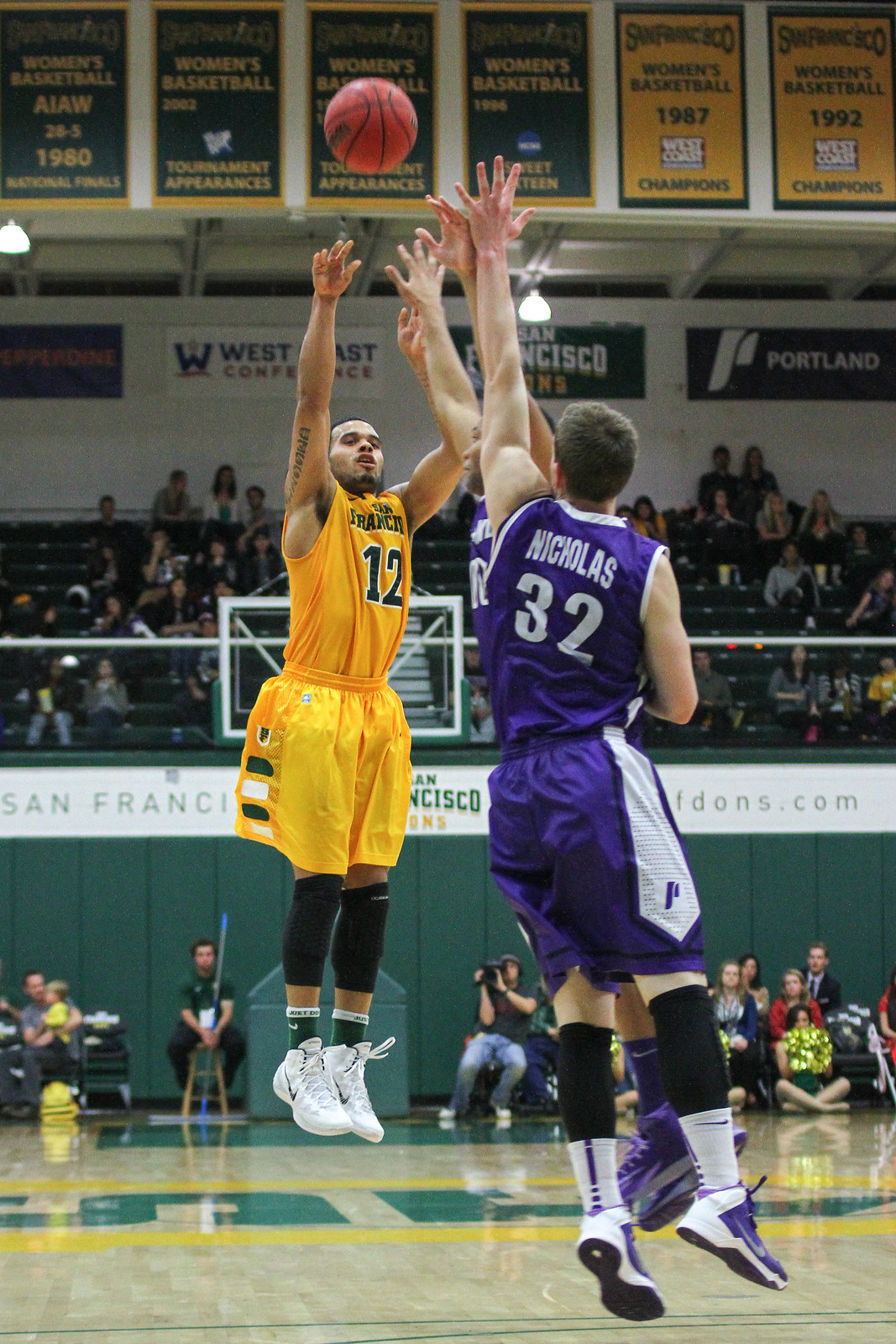The photograph captures an intense moment during a high school or college basketball game, where a player in a yellow jersey with the number 12 is seen midair just after releasing a shot. He is sporting white shoes and black knee braces, and is surrounded by two players in blue and white jerseys attempting to block his shot. One of the defenders, number 32, has “Nicholas” written on his uniform. The basketball is suspended between the players' outstretched hands. The gymnasium features a light wood sports floor with green and gold lettering, while the backdrop includes a tall green wall and stands filled with cheering spectators. Banners showcasing past tournament championships, predominantly green and gold, hang above the crowd. Additionally, someone with an old-fashioned camcorder is visible among those seated at the base of the wall, capturing the action.